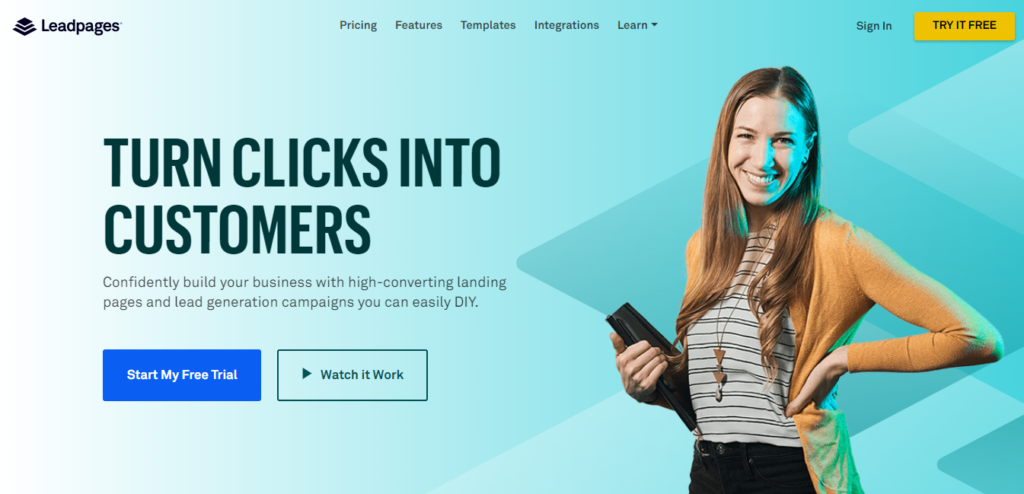The image showcases the homepage of a website named "Lead Pages," dedicated to providing templates. At the top left, the website's title, "Lead Pages," is prominently displayed beside a logo featuring a stack of papers arranged in a pyramid-like structure. Centrally positioned at the top are five navigation categories: "Pricing," "Features," "Templates," "Integrations," and "Learn." 

Located at the top right are two interactive sections; a yellow box labeled "Try It Free" in black text, and next to it, the "Sign In" link. Dominating the middle right portion of the image is a photograph of a woman with a fair complexion and long, light brown hair cascading to her chest. She appears confident with her left hand resting on her waist and her right hand holding a device or folder. Her attire includes a white and black striped shirt, an orange jacket, dark trousers, and a necklace composed of a series of interconnected triangles. Her elegant stance and focused gaze convey professionalism and approachability, complementing the website's theme.